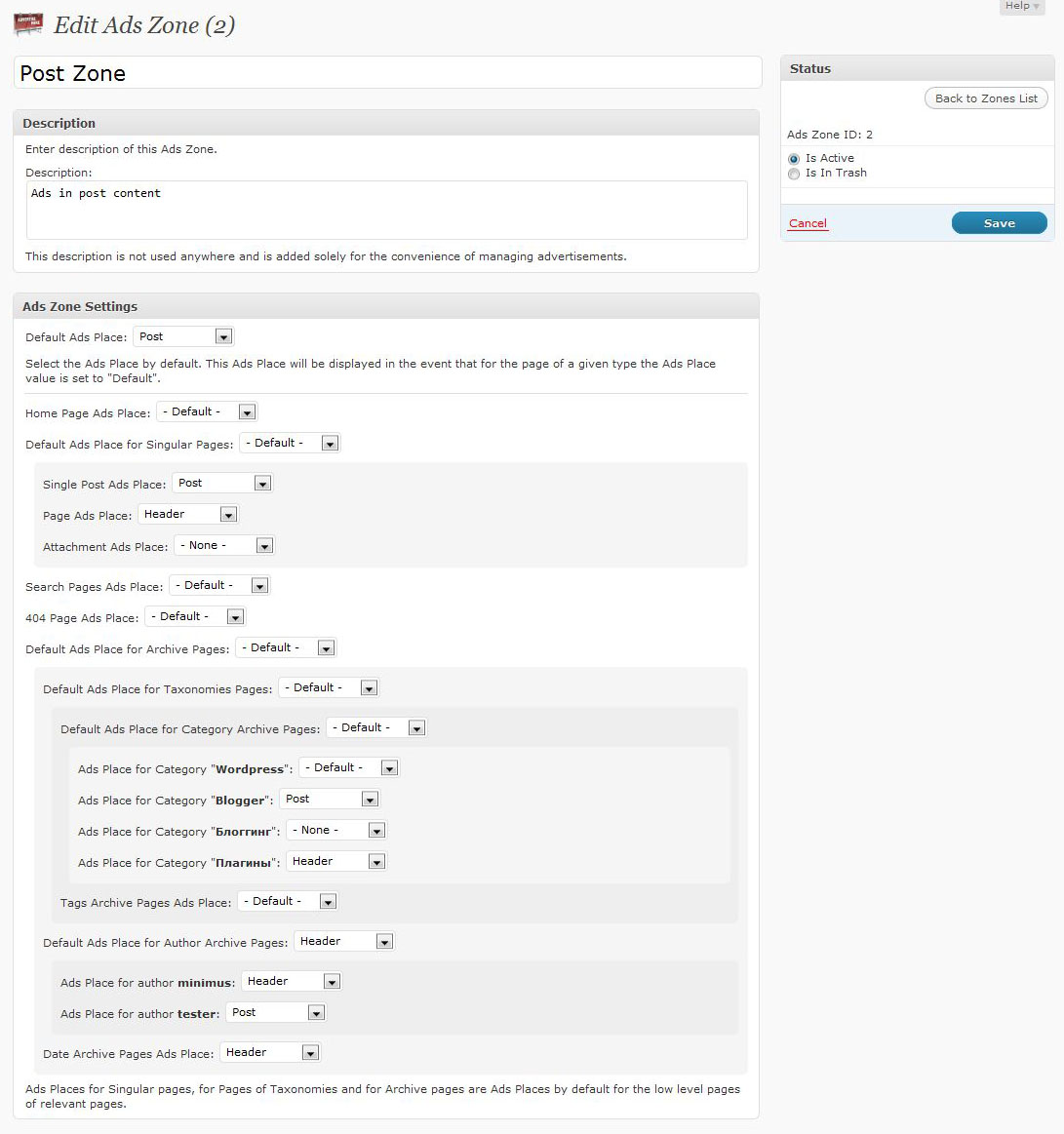This detailed caption describes the interface of a digital tool used for managing advertisement zones on a blogging platform. 

---

This image showcases a user-friendly interface designed for editing advertisements on a blog. At the very top, the tab is labeled "Edit Ad Zone," followed by a "Post Zone" section underneath it. This section allows users to manage and describe ad content, although this description is not used within the actual ad itself; it is solely for organizational purposes. 

The interface offers various settings for manipulating ad zones. It lists default ad placements where users can select the default ad position, which will be displayed when a specific type of page is viewed. For instance, the home page, singular pages, or search pages all have default ad placements. 

There is a comprehensive list of options for ad placements including single post pages, ad pages, attachment pages, search pages, and even 404 error pages, all of which are initially set to default. Furthermore, users have specific settings for WordPress and the ability to adjust the ad placement for categories and headers, with different language options like Russian available. 

On the top right of the interface, a help button and a status box are present. Users can also navigate back to the zones list. The current ad zone is shown as active, and users have the options to save their settings or cancel any changes made. This tool is assumed to be particularly useful for individuals managing advertisements on their blogs, allowing them to have a comprehensive control over their ad placements and settings.